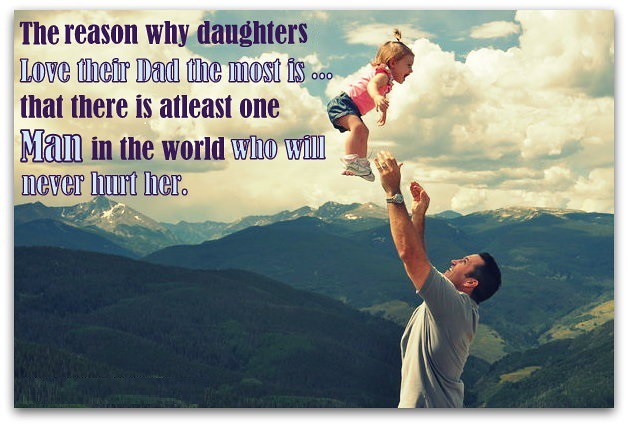In this bright and sunny image, a strong, dark-haired man wearing a grey shirt is joyfully tossing his baby daughter into the air. Her face is lit up with a radiant, happy smile as she soars, her blonde hair tied in a small ponytail on top of her head. She is dressed in a pink shirt, blue shorts, and white sneakers with pink and teal accents. In the background, a majestic grassy mountain range stretches out under a clear blue sky filled with beautiful puffy white clouds. Text in alternating dark blue and light purple lines runs along the upper left-hand corner of the image, reading: "The reason why daughters love their dad the most is that there is at least one man in the world who will never hurt her." The landscape and the joyful interaction between the father and daughter create a heartwarming scene, bathed in sunshine.